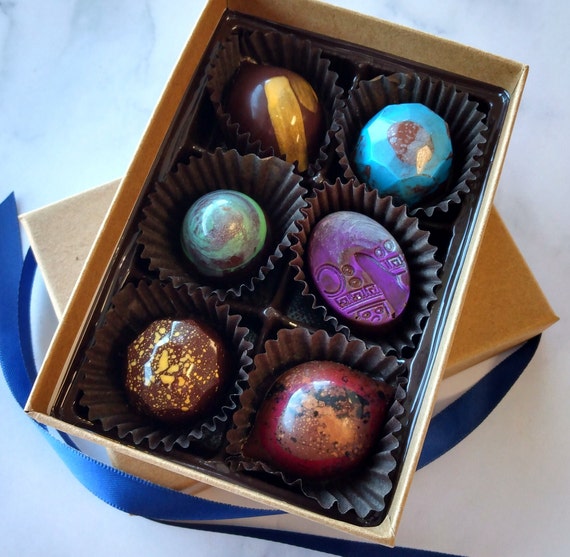The image depicts a gourmet box of chocolates arranged diagonally. The box contains six uniquely designed chocolates, arranged in two columns and three rows, and it rests atop the box lid which is also oriented diagonally but at a sharper angle. A blue ribbon, likely the original wrapping, lies besides. Each chocolate is housed in dark brown, cupcake-like wrappers. 

Starting from the top left: the first chocolate is dark brown with a yellow stripe. The second is baby blue marbled with chocolate color and hexagonal in shape. The middle row's left chocolate is green marbled with brown, resembling a small planet, while the right one is oval, purple, with embossed details. The bottom row features a dark brown truffle dotted with yellow on the left, and a red chocolate marbled with orange and black on the right. All chocolates are shiny, artistic, and appear to be a product photo, emphasizing their luxurious and sophisticated appearance.